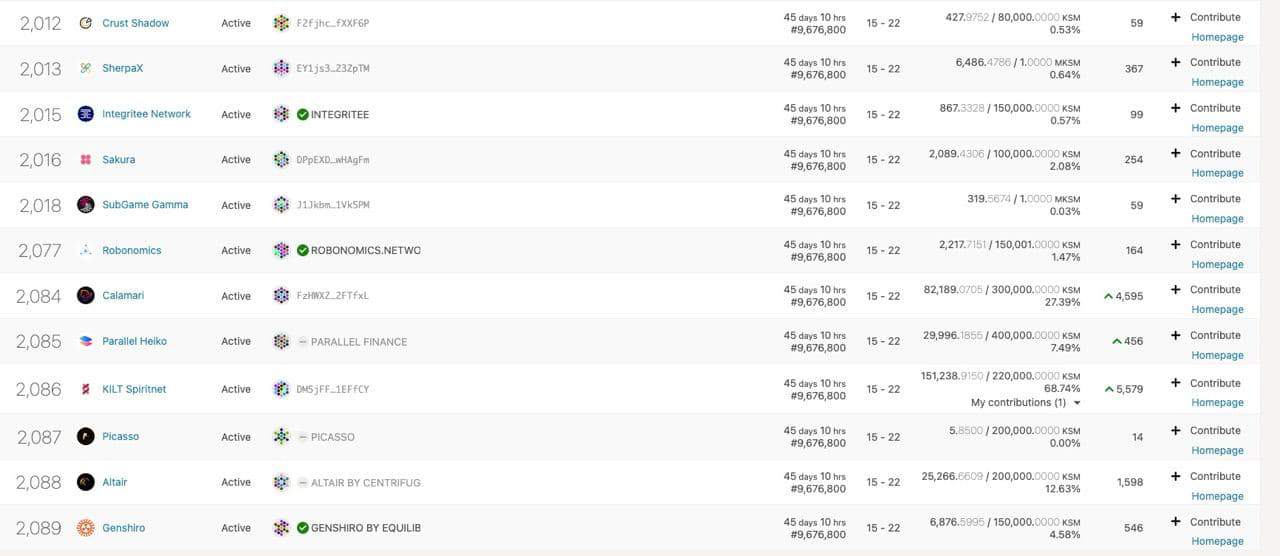*On a horizontal rectangular sectioned page with alternating white and light gray lines:*

1. **2012:**
   - Icon: [Unclear, possibly representing 'Crush Shadow']
   - Status: Active
   - Statistical details: 
     - Duration: 45 days, 10 hours
     - Numeric value: 9,676,800
     - Range: 15-22
     - Metrics: 427 / 80,000
     - Percentage: 0.53%
   - Additional Information:
     - Number: 59
     - Option: Plus Contribute
     - Link: Homepage (highlighted in blue)

2. **2013:**
   - Project: Sherpa X
   - Icon: [Logo]
   - Status: Active